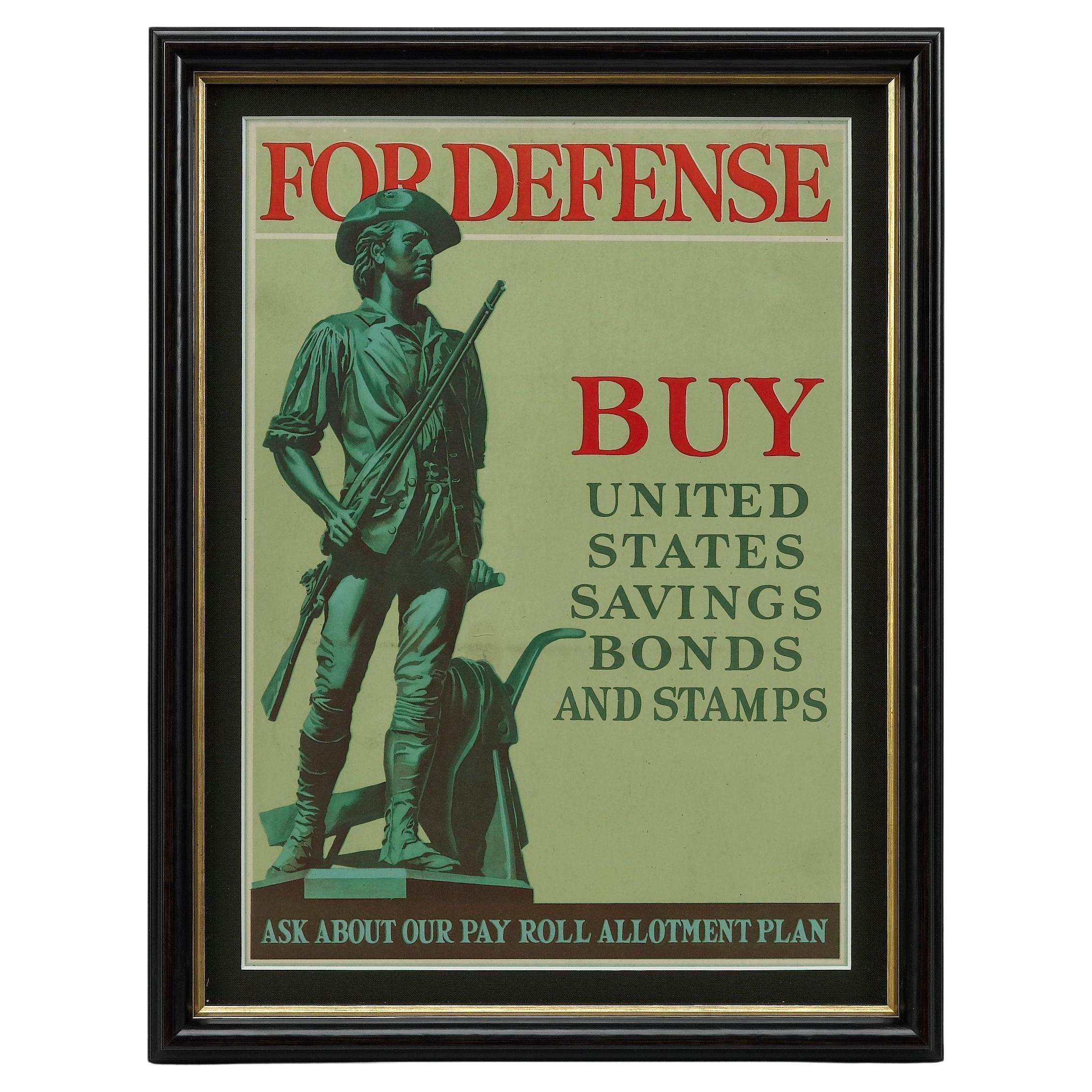The image is a framed advertisement promoting United States Savings Bonds and Stamps. The ad is encased in a black wooden frame, relatively thin and lined with gold on the inside. Surrounding the advertisement is black matting. The poster itself has a light green background, possibly sage or army green, and features an older style American soldier, likely from the 18th century American Revolution. The soldier, positioned on the left, is depicted wearing a distinctive hat folded up at the side, a deerskin shirt with fringe, leather pants, and moccasin-like boots. He carries a rifle in his right hand. 

At the top of the poster, in bold red capital letters, the words "FOR DEFENSE" stand out. Below it, separated by a white line, the word "BUY" is prominently displayed in red capital letters as well. Further down, in a darker green color, is the phrase "United States Savings Bonds and Stamps," arranged vertically. At the bottom of the poster, in lighter green horizontal capital letters, it reads, "Ask About Our Payroll Allotment Plan." The poster exudes a patriotic and historical aura, emphasizing defense and financial savings for the nation.